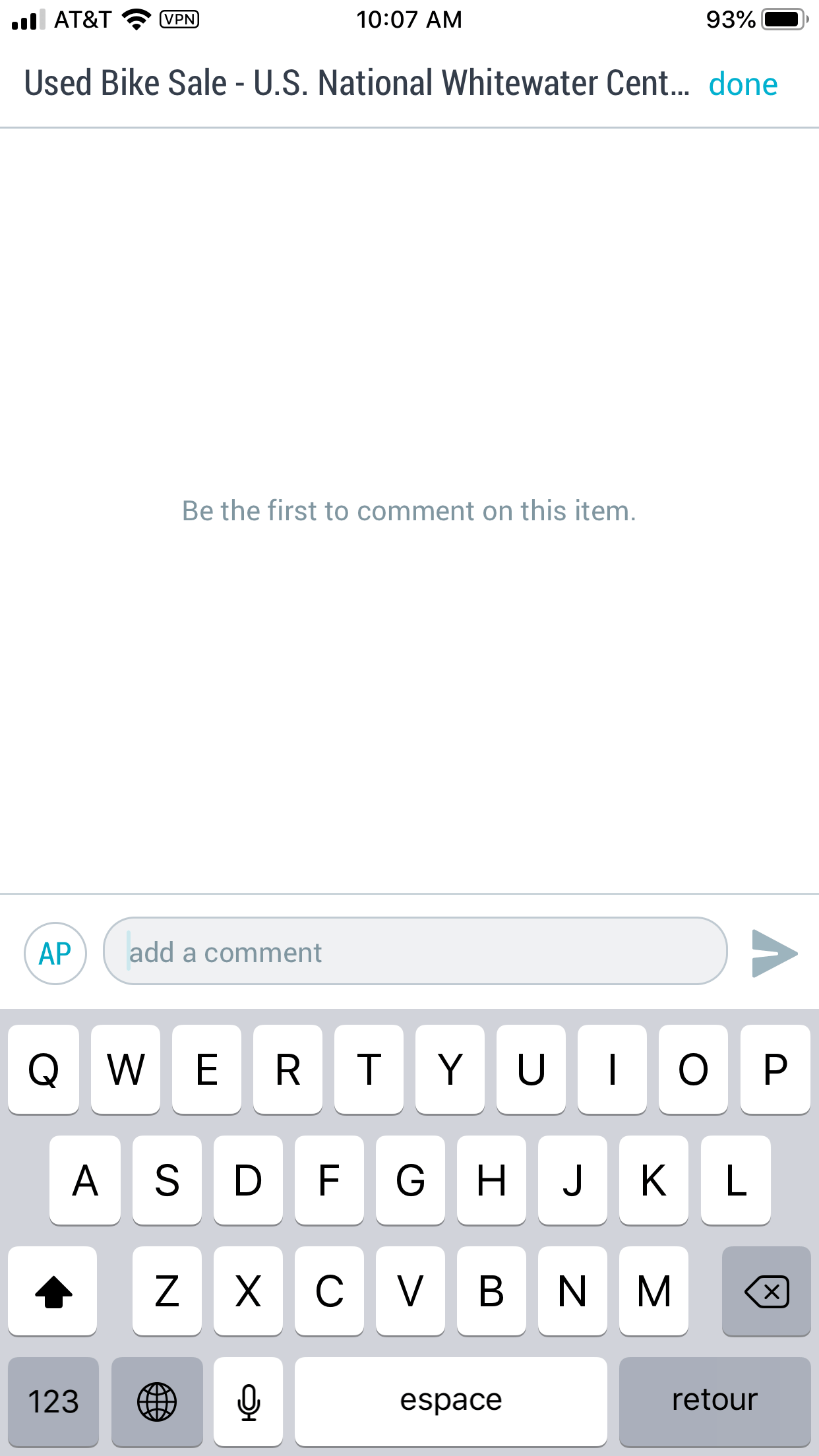In this image, a phone screenshot displays a partially filled signal bar in the upper left corner, indicating three out of four bars of connectivity. Next to it, "AT&T" is visible, followed by a Wi-Fi symbol and a rectangle indicating "VPN." The time, "10:07 AM," is centered at the top of the screen. 

On the upper right, a battery icon shows 93% charge. Below that, a title reads "Used Bike Sales - U.S. National Whitewater Center..." with "Done" appearing in blue next to it. 

Centered on the screen, a prompt reads, "Be the first to comment on this item." Below that, a line separates it from the "Add Comment" section, which features a long oval text box for input. On the right of this text box is a right-pointing arrow. On the left of the text box, an icon with the letters "AP" is circled and highlighted in blue. 

At the bottom of the screenshot, the phone's keyboard is visible, including symbols for a microphone and a globe.